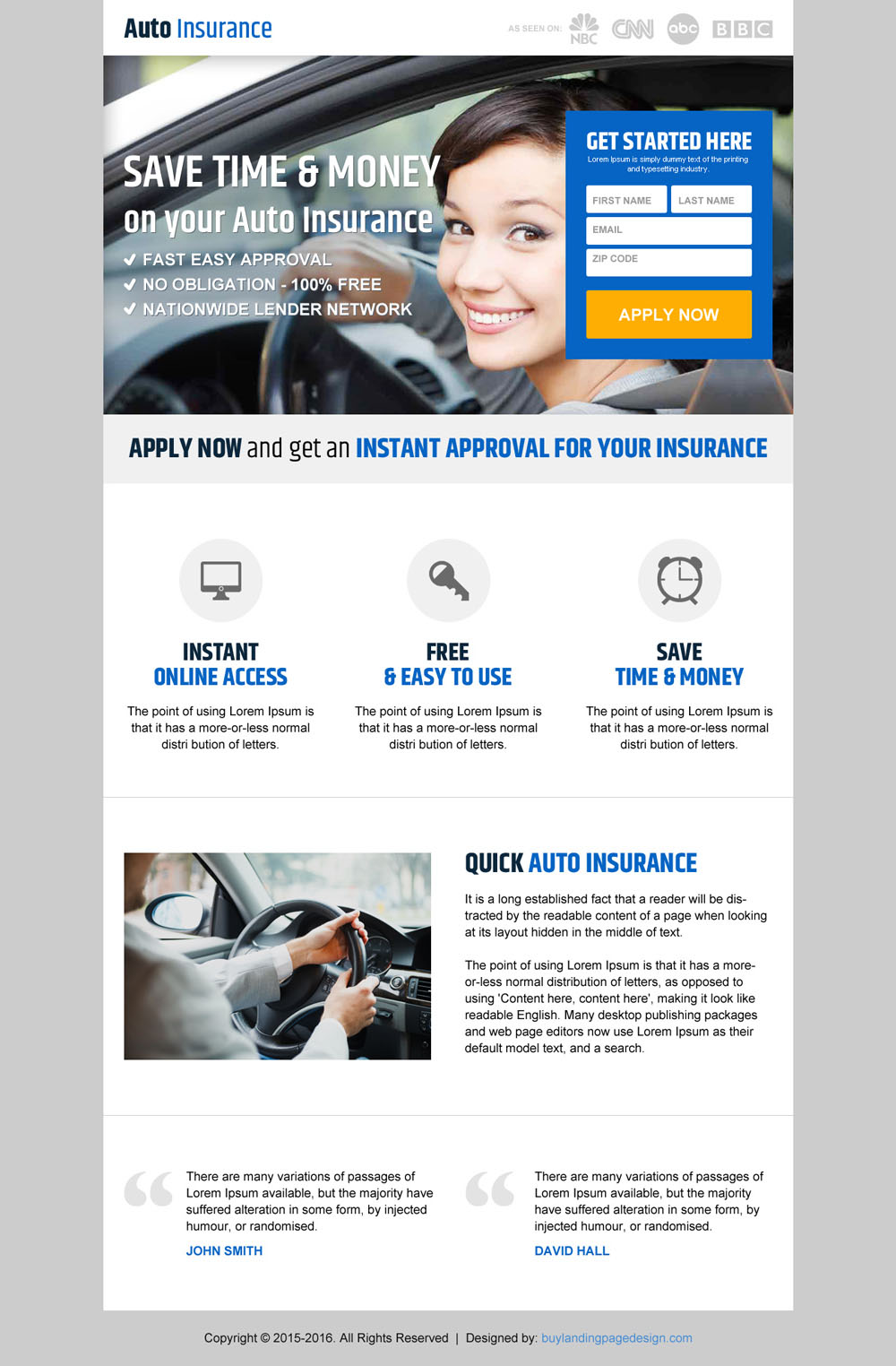The image features a webpage designed to promote auto insurance services. 

**Header**:
- *Top Left*: The text "auto insurance" is prominently displayed, with "auto" in black and "insurance" in blue.
- *Top Right*: Iconic logos of renowned news providers including CNN, ABC, and BBC.

**Main Section**:
- *Heading*: "Save time and money on your auto insurance" followed by benefits listed in short phrases: "Fast, easy approval, no obligation, 100% free, nationwide lender network."
- *Background Image*: A cheerful man is depicted driving a car, smiling, symbolizing satisfaction and ease.
- *Sign-in Box (Right Side)*: A blue box with white text titled "Get started here." The form requires entries for first name, last name, email, and zip code. Below this, an orange button labeled "Apply Now" is present.

**Footer**:
- *Central Section*: A call to action with the instructions "Apply now and get an instant approval for your insurance." The phrase "instant approval for insurance" is in blue, while the rest is in black. Below, there are three highlighted steps:
  1. *Instant Online Access*: Accompanied by placeholder text explaining the use of Lorem Ipsum.
  2. *Free and Easy to Use*: Also followed by a Lorem Ipsum explanation.
  3. *Save Time and Money*: Reiterates the Lorem Ipsum placeholder text.

- *Bottom Left*: User reviews section with text: "There are many variations of passages of Lorem Ipsum available. However, the majority have suffered alternation in some form by injected humor or randomized words." Authored by John Smith.
- *Bottom Right*: Another set of reviews stating: "There are many variations of passages." This review, similar to the previous one, is concluded by David Hall.

**Footer Text**:
- "Quick auto insurance" prominently displayed.

This dense and detailed layout presents a clear, attractive interface designed to encourage users to apply for auto insurance swiftly and confidently, bolstered by trust-building elements and user testimonials.